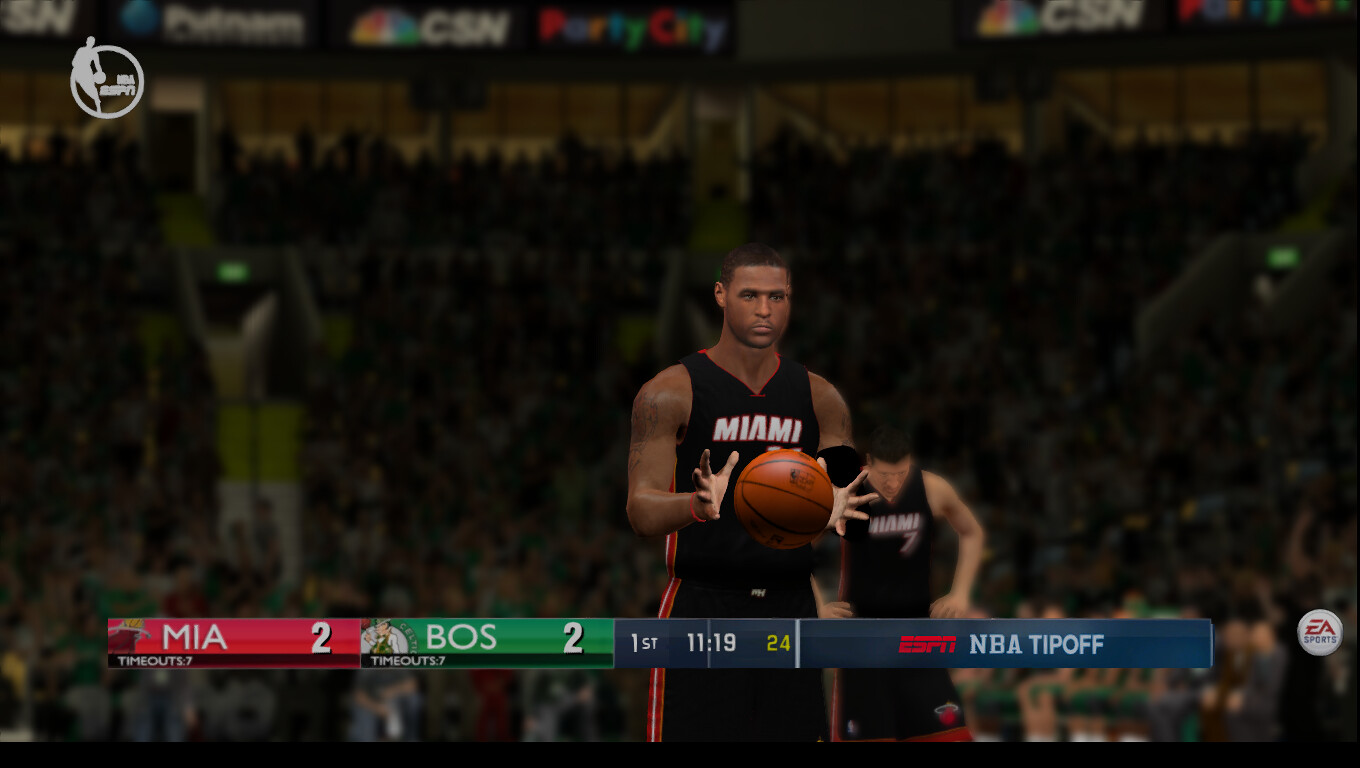The image appears to be a screenshot from an NBA video game, showcasing a key moment of the action. Dominating the scene, a black basketball player from the Miami Heat is about to catch the ball. He stands at the center, wearing a black uniform with red and white trim, emblazoned with the word "Miami" in white letters across his chest. His hands are extended in front of him, elbows bent and palms nearly touching the basketball that hangs in the air between them. The player has short black hair and a focused expression as he zeroes in on the ball. 

In the background, a blurred white player with his hands on his hips surveys the game. The dark, indistinct backdrop suggests a stadium filled with spectators, adding to the game's immersive atmosphere.

The on-screen display provides further context: in the upper left corner, an NBA ESPN logo is visible. At the bottom, a score display with a red backing shows "MIA" for Miami with a score of 2, and a green rectangle for "BOS" representing Boston, also with 2 points. The first quarter has 11 minutes and 19 seconds remaining, with 24 seconds on the shot clock. Additionally, it reads "ESPN NBA Tip-off" alongside the EA Sports logo on the right.